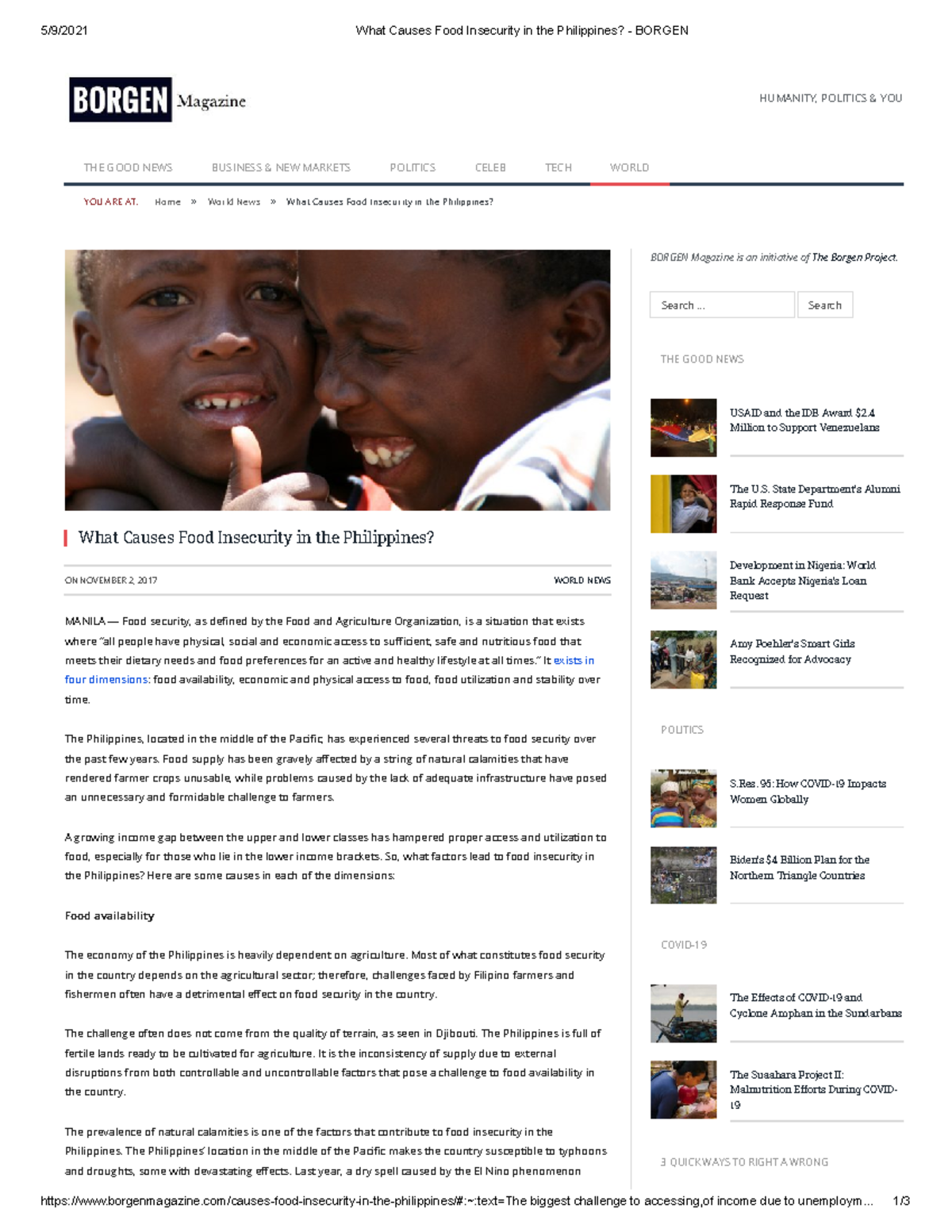The image depicts an article from Borgin Magazine's website, dated May 19, 2021. The headline at the top center reads "What Causes Food Insecurity in the Philippines?" Below the Borgin Magazine logo on the left, a menu is visible listing sections such as The Good News, Business and New Markets, Politics, Celeb, Tech, and World, separated by a black bar. Underneath the menu, it indicates that the user is on the current article page. 

In the main content area, there's a heartwarming close-up picture of two young boys. The boy on the right is looking to the left, while the boy on the left is facing the camera with a thumbs-up gesture. The emotional image emphasizes the human impact of the article's topic, food insecurity in the Philippines.